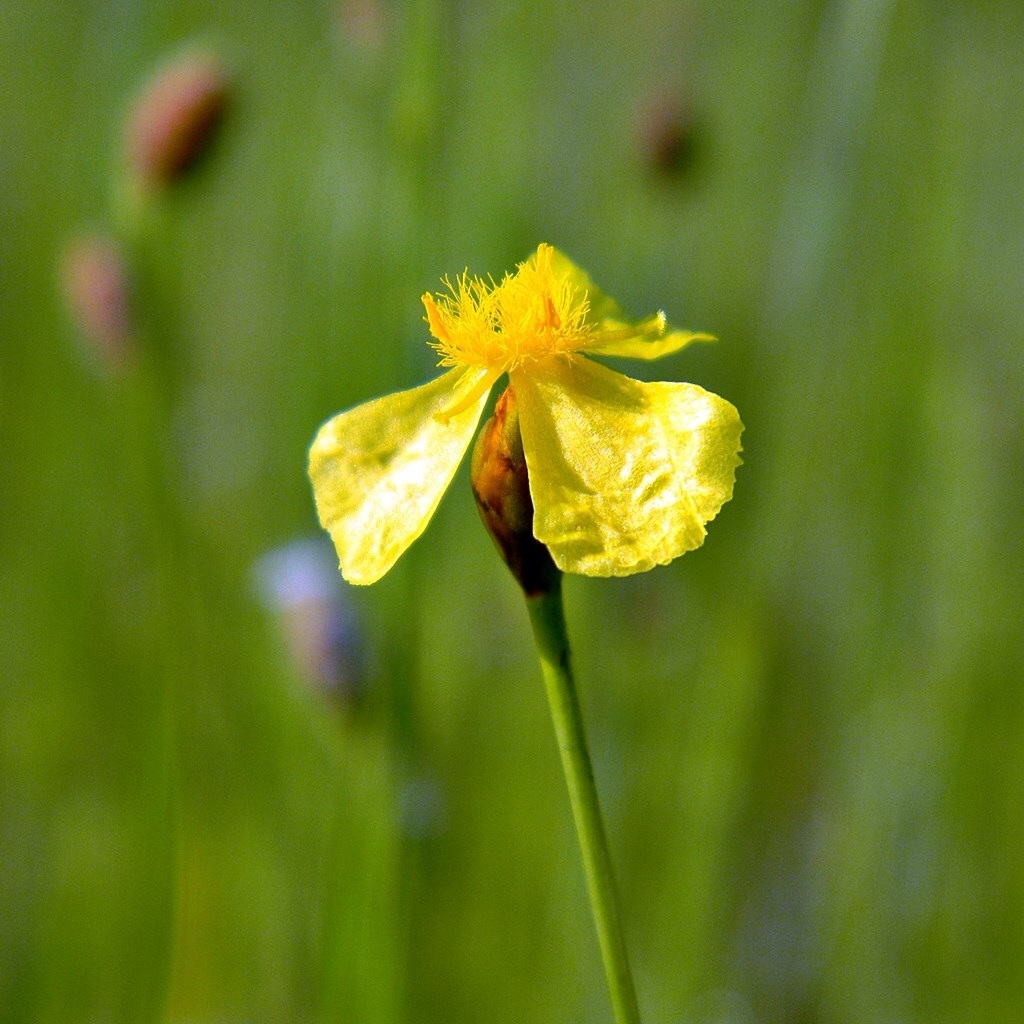This close-up color photograph captures a striking yellow flower with three small, slightly ragged petals that are beautifully illuminated by sunlight. The petals are curved with rounded, frayed edges, and their vibrant yellow hue stands out vividly. At the heart of the flower, a fibrous and golden-yellow center extends upward, adding texture and complexity to the delicate bloom. The flower is supported by a long green stem and appears to be past its prime, yet it retains an undeniable natural beauty. The background of the image is a blurred expanse of green, possibly a meadow or field, with hints of red and purple plant life softly visible, enhancing the focus on the central flower. The overall effect is a mesmerizing snapshot of nature, with every artistic element directing attention to the bright, central flower.